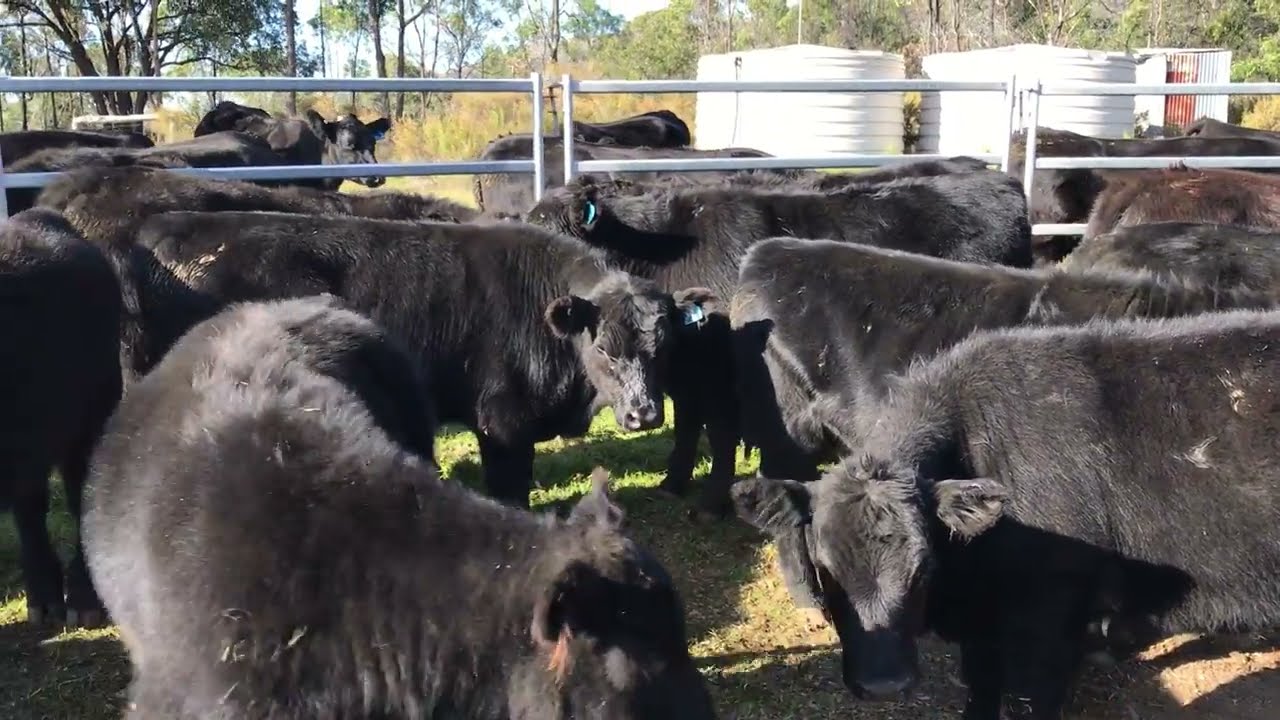In this outdoor photograph taken on a sunny day, a herd of approximately 13 black cattle is gathered in an open pen surrounded by a gray, metal fence. The ground within the pen is a mix of straw and sparse grass, with some cows showing signs of having lain in the dirt. Their coats are dotted with patches of brown dirt, particularly on their hindquarters. Many of the cattle sport blue tags on their ears. The scene is set against a backdrop of lush, green trees and bushes, indicating a wooded area beyond the enclosure. The sunlight casts long shadows of the cattle, reinforcing the impression of a bright day. In addition to the natural scenery, the upper left corner of the image reveals a silver, partially rusted metal outbuilding or container. The cows appear relaxed, with most facing to the right, and a few even seem to be captured mid-movement. The photographer's shadow is visible in the lower left center of the image, suggesting the light source is positioned behind them. Overall, the healthy, robust cattle in this serene farm setting exude a sense of calm and contentment.